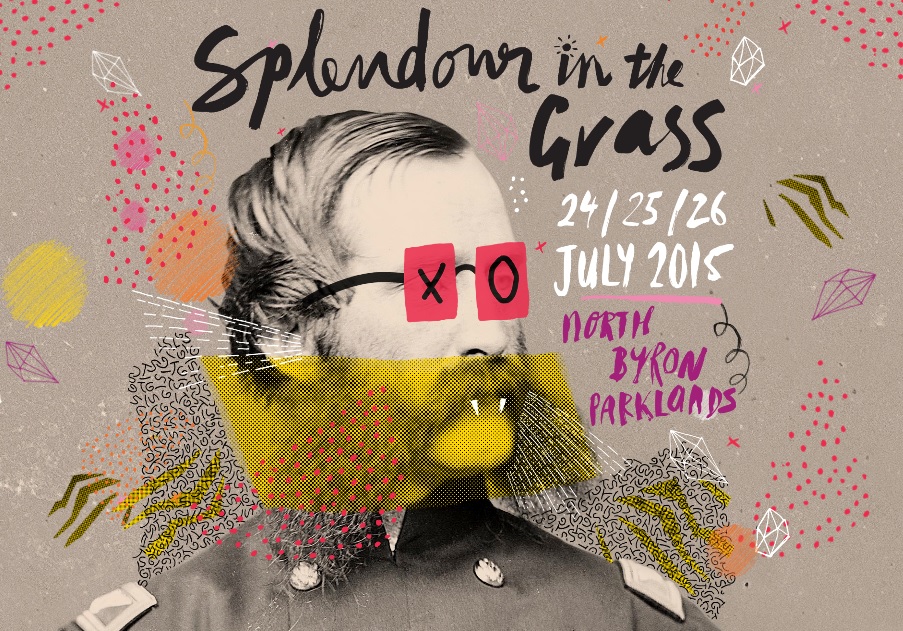The image is a vibrant and eclectic poster centered around a black-and-white photograph of a Confederate soldier, who sports a short haircut and a broad mustache. Overlaying his face are whimsical and surreal elements: red boxy eyeglasses with one lens marked by an "X" and the other by an "O," drawn white fangs protruding from his mustache, and a yellow swath across his jaw and chin. The soldier's uniform features a gray shirt with white buttons and epaulettes, further enhancing his historical look. The backdrop of the poster is an artful montage with a neutral grayish-brown tone, adorned with a riot of colors including reds, purples, greens, yellows, and pinks.

At the top, against a shifting white-purple background, bold black letters announce "Splendor in the Grass." Just below, in white text, are the dates "24, 25, 26 July 2015," with "North Byron Parklands" written in purple underneath. The surrounding decorative elements include red dots, diamond sketches, and larger yellow and pink circles, adding to the dynamic and layered imagery. Overall, the poster blends historical and modern artistic elements to create a vivid, eye-catching composition.